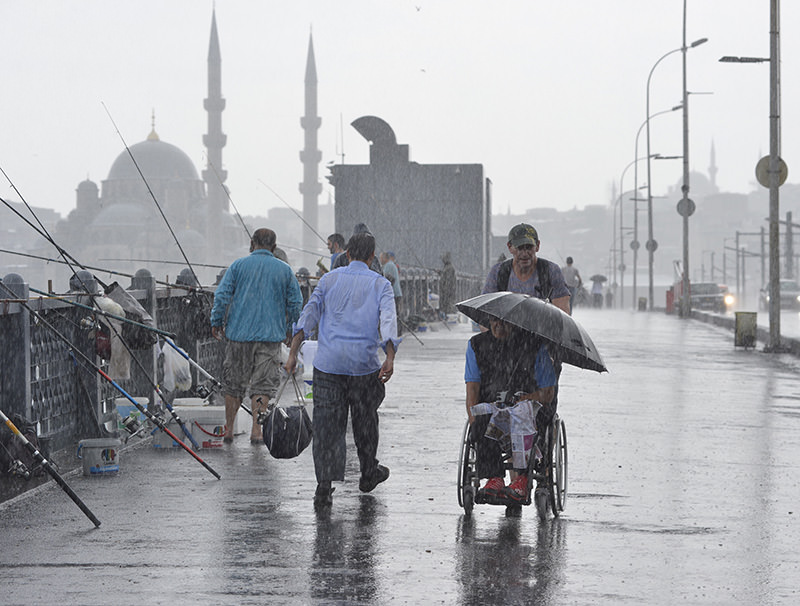A vibrant, full-color square photograph captures a lively scene on a rainy day, taking place outdoors during daylight with natural light. The setting is an expansive stone-paved bridge adorned with a gray stone railing on the left, hinting at a location in the Middle East or India, characterized by domed roofs and temple-like structures with tall spires in the distant background. The wet pavement, glistening with puddles and reflecting the people, suggests recent rain.

Along the left side of the bridge, numerous fishing poles are propped up against the railing, alongside bait and tackle buckets, though there are few anglers present. Towards the center right of the image, a man in a collared shirt is pushing another man in a wheelchair, who is holding a black umbrella—the only one in the scene, despite the wet environment.

To the right, a bustling road with cars approaching the viewer adds to the dynamic nature of this foreign urban landscape. Scattered across the bridge are various pedestrians: two men in blue shirts walk away from the camera, one carrying a bag, and a mix of others, including a woman, all braving the rain without umbrellas. The scene captures the blend of daily life, resilient against the elements, in a distinctly non-Western setting.